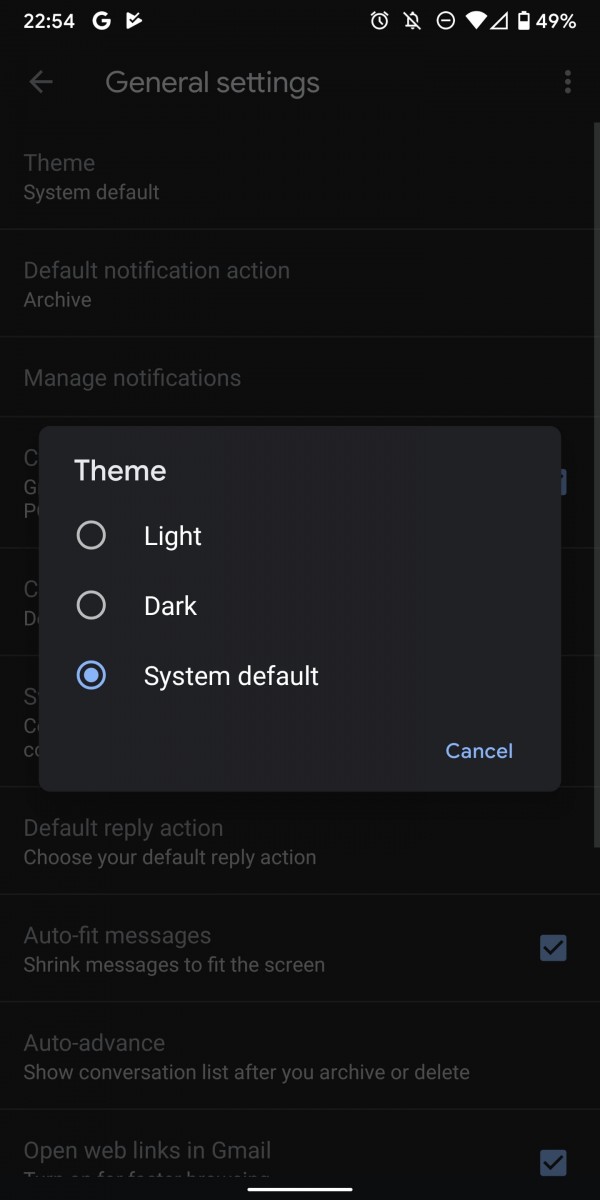This is a detailed screenshot of a smartphone displaying its General Settings page on a black background. The status bar at the top of the screen shows the time as 22:54 in white text, with a Google 'G' icon and a triangle with a check mark next to it, indicating system notifications. To the right, various icons represent the active alarm, silent mode, Do Not Disturb mode, data or Wi-Fi connectivity, and battery percentage.

The main section of the screen highlights the "Theme" settings, which is set against a muted gray background. The active selection area is a dark gray rectangle in the center of the screen. In this area, white text options are displayed with their respective selection indicators: “Theme” (unselected), “Light” (unselected), and “Dark” (selected). The “Dark” option is noted as the "System Default" with a filled selection circle. On the lower right corner of this dark gray section, there is a light blue "Cancel" link, providing an option to discard any changes.